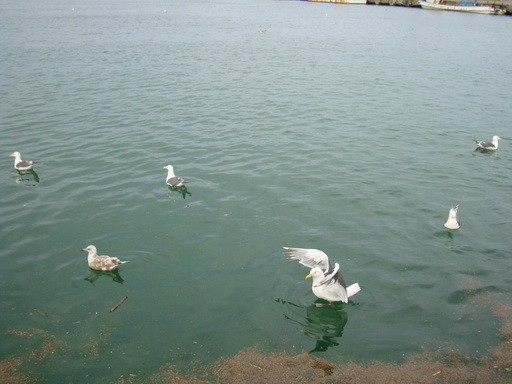This outdoor daytime photograph captures a lake scene with calm greenish water and six white seagulls with gray wings. The water's color transitions from a grayish top to green and finally brownish at the bottom, possibly due to brown algae or scum floating near the seagulls. Most of the seagulls are peacefully floating, their reflections casting a greenish tint in the water, while one seagull appears to be raising its wings, either about to take off or just flapping. In the upper right-hand corner, the faint outlines of buildings or a pier are visible, along with a long white boat on the water. The left side of the water is perceptibly greener compared to the slightly bluer right side. The entire composition focuses on the water and the seagulls, with no people or sky visible in the image.